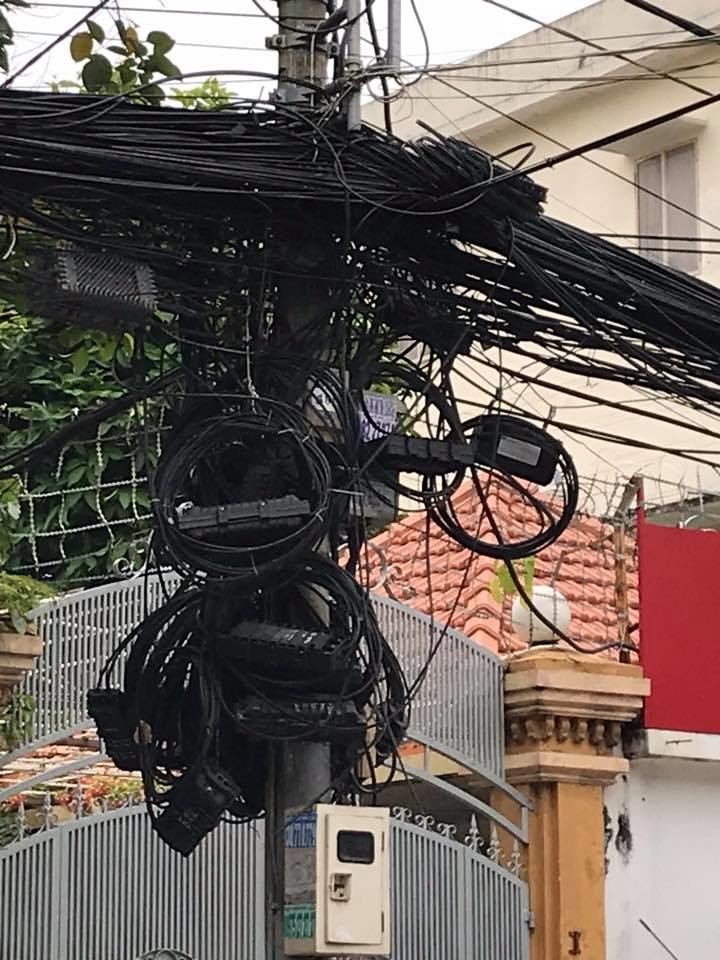In the image, an ornate white building with a rich sculpted entrance stands in the background, giving an impression of grandiosity despite its somewhat run-down appearance due to the cluttered arrangement of black cables. Dominating the foreground is a grey pole, heavily wrapped with an overwhelming number of black wires that seem tightly coiled and bound around it, some of which extend outwards and crisscross in multiple directions. This intricate mess of cables is so densely packed that it includes various labeled boxes and other telecommunication attachments. Surrounding the area is a tall, silver-grey fence with detailed French-style embellishments at the top, partially hidden by vibrant green foliage that creeps into the scene. Additional elements in the backdrop include a beige house and a house with a red clay roof, which contrast sharply with the dark cables, further emphasizing the complex wiring against the lighter background. The overall composition of the image, taken outdoors with a regular camera, conveys a striking contrast between the structured elegance of the buildings and the chaotic entanglement of the numerous black wires.